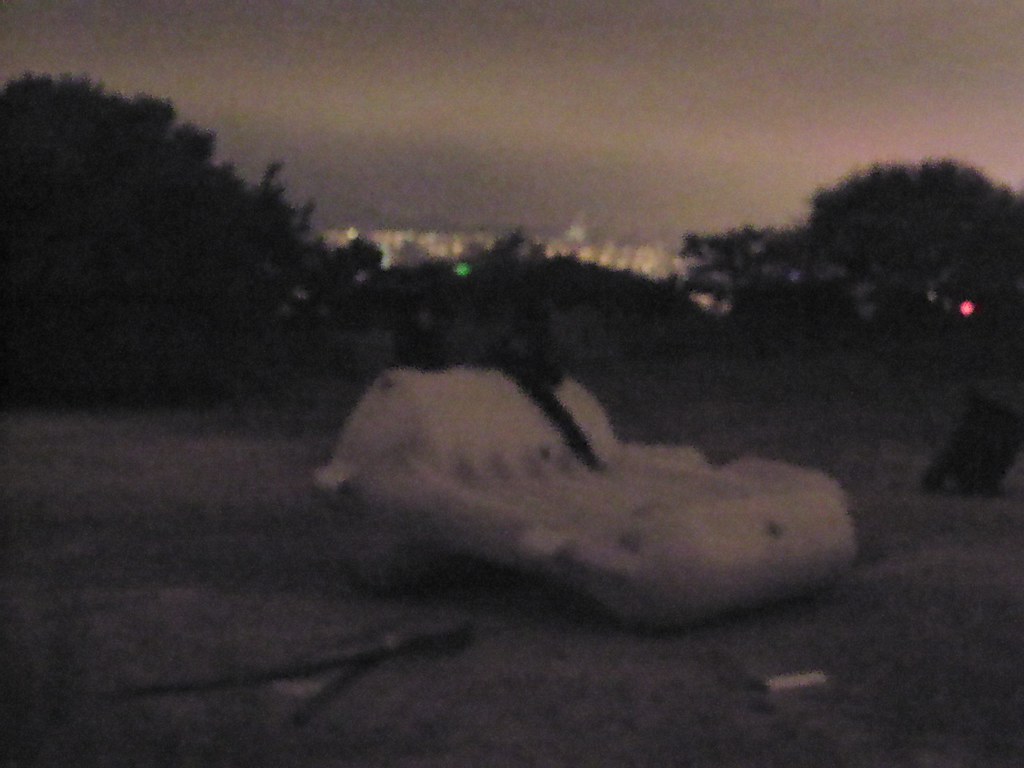This grainy, sepia-toned nighttime photograph captures a distant, brightly lit cityscape against a dark sky, softly illuminated by light pollution. In the foreground, the image reveals a flat, white object with rounded edges—resembling either a vehicle or a seat—resting on a grassy or dirt-covered terrain. Amidst the muted backdrop, some trees are discernible on the horizon, situating the scene on a hill that overlooks the sprawling urban glow below.